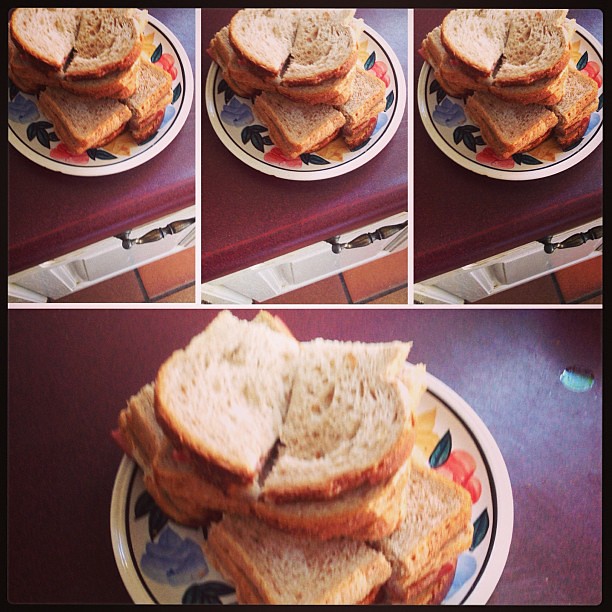The image depicts a collage of four photographs, arranged with three equal-sized rectangles on the top and one long rectangular photo on the bottom, all focused on a stack of sandwiches on a intricately painted white plate. The plate features a floral wreath design with broad brush strokes, depicting flowers and leaves in blues and reds, creating a hand-painted look. Each photo provides a progressively closer view of the sandwiches, which are made with toasted white bread cut into various shapes—some in quarters and some diagonally—arranged on the plate. The bottom photograph offers an overhead shot of the sandwiches, on a maroon countertop. In the top left corner of the bottom photo, a small drip of liquid is visible on the counter. The setting includes a white drawer with a bronze pull handle and a terracotta-colored tiled floor with gray grout, adding to the overall scene's 1980s aesthetic.